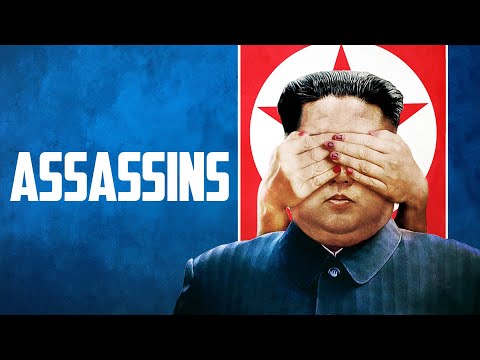The image is a humorous promotional piece for a movie or event, satirizing a real-life politician, specifically the leader of North Korea, Kim Jong-un. The top and bottom of the image feature solid black borders. The main background is predominantly blue with a gradient, smoky pattern of light and dark blue hues. On the left side, the word "Assassins" appears in bold, all-caps white text. 

Positioned to the right, there is a close-up of Kim Jong-un from shoulders upwards. He is wearing a blue striped button-up shirt with long sleeves, and his glossy, heavily gelled hair is brushed back. His expression is notably unhappy, sporting a pronounced frown. Covering his eyes are two hands, adorned with red-painted nails, which seem to belong to a different person. 

Behind Kim Jong-un is a red banner featuring a white circle with a red star at its center, with three points of the star visible. The overall composition creates a striking contrast between the blue background and the vivid red elements, amplifying the satirical tone of the image.